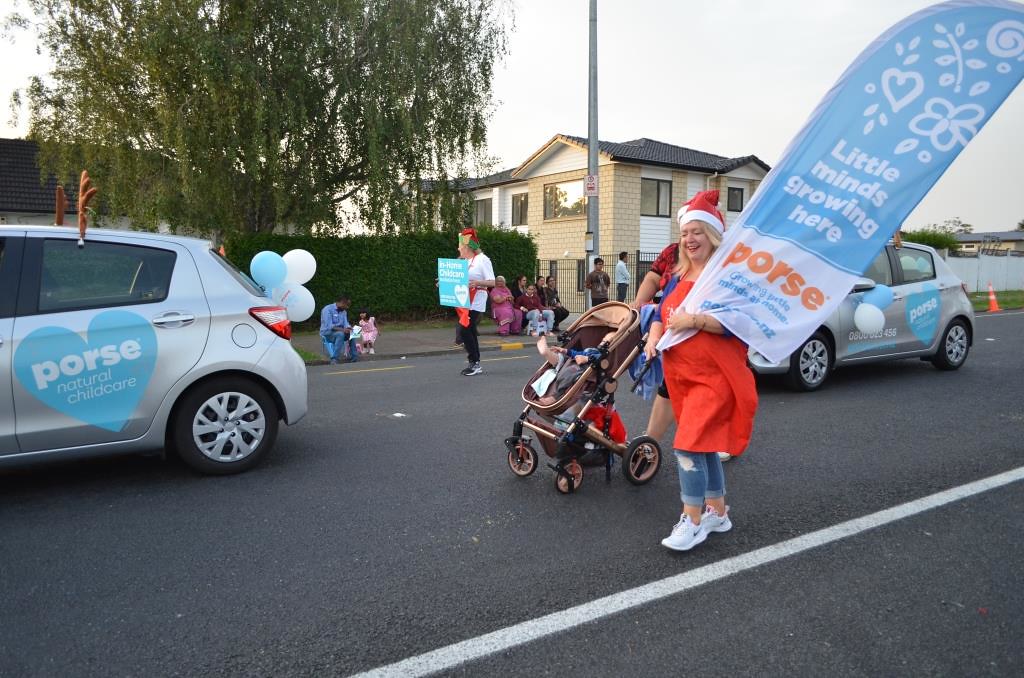The image captures a festive yet poignant funeral procession moving down an asphalt street. Central to the scene is a smiling woman with blonde hair and closed eyes, wearing a Santa Claus hat, a long red t-shirt, blue jeans, and white sneakers. Over her blue shirt, she wears a red apron. She proudly carries a large, blue-and-white sign adorned with drawings of hearts, flowers, and teardrops, stating "Little Minds Growing Here." Below this, the name "Porsche" is written in vibrant orange letters on a white background.

Accompanying her are several people, including a man pushing a baby carriage. The procession is flanked by two small silver cars, each adorned with white and blue balloons and the inscription "Porsche Natural Child Care" with a heart symbol on the door. Positioned between the cars, the woman stands out as a key figure in this heartfelt gathering.

In the backdrop, a two-story gray brick house with white paneling and a black ranch-style roof is partially obscured by a large willow tree on the left. The scene includes additional elements such as a prominent metal post, shrubbery, and a telephone pole, set against a mostly white sky. A person in the background interacts with a child, and others are seen congregating, adding to the communal atmosphere of this solemn yet celebratory event.